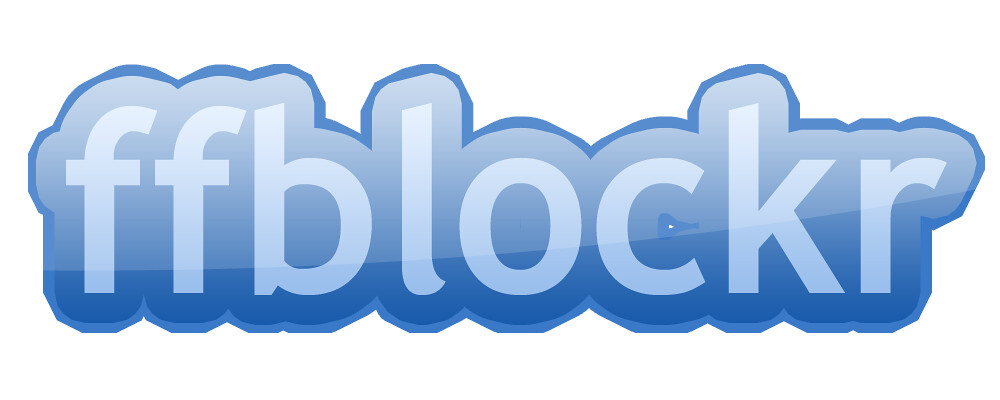The image prominently features a computer-generated logo set against a stark white background. At the center of the image, the text "FFBLOCKR" is displayed in light blue, lowercase letters. The letters are encased in a motif of varying shades of blue that form a soft, cloud-like outline around the text. Beyond this cloud-like encasement, a darker blue border provides additional contrast. The overall design gives the impression of a modern company logo or a graphic element that could be used for digital branding, such as on a website or a business card. The clean and simplistic background enhances the focus on the logo, ensuring that "FFBLOCKR" is the central visual element without any other text or hashtags to distract from it. The balanced composition and meticulous color coordination contribute to the logo’s sleek and professional appearance.